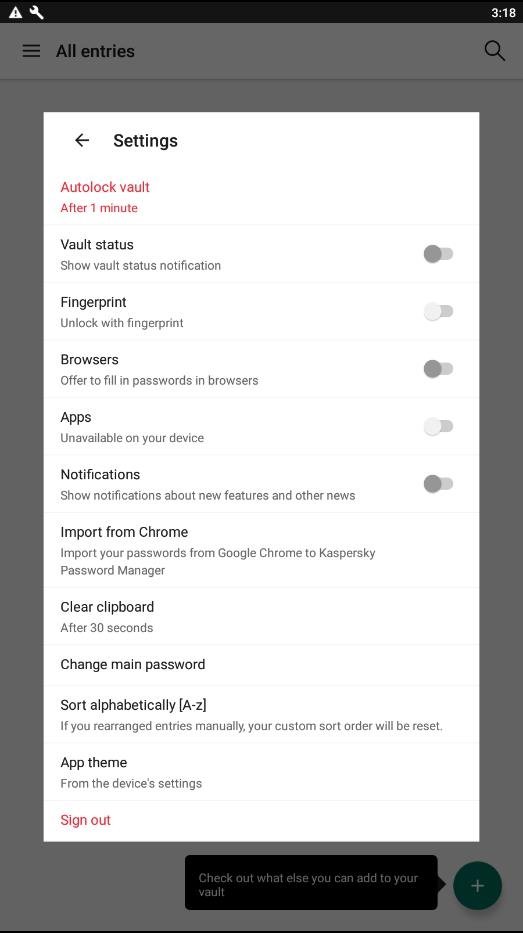Here's a detailed, cleaned-up descriptive caption for the image:

---

The screenshot depicts a phone's settings menu, within the configuration settings of a password manager. A white popup box is centered on the screen, titled "Settings" at the top with a back arrow on the left. Below the title, the first option displayed is "Auto Lock Vault," highlighted in red, set to activate after one minute. Next is "Vault Status," currently deactivated as indicated by a slider positioned to the left. 

Following this, there's a "Fingerprint" option to enable fingerprint locking, which is also disabled with a left-positioned slider. Below it is the "Browser" setting, designed for automatic password entry in browsers, again showing a deactivated status. The "Apps" section follows, marked as unavailable on the device, likewise toggled off.

Further down, the "Notifications" feature is listed, which can be enabled by sliding to the right, though it is currently off. The options for "Import from Chrome" are included, allowing the user to import passwords from Google Chrome to Kaspersky Password Manager. Additionally, there is a "Clear Clipboard" feature set to clear the clipboard after 30 seconds.

Users can also "Change Main Password" and have the option to "Sort Alphabetically," with a note that manual reordering of entries will reset any custom order. The menu ends with "App Theme" and "Sign Out" options in red, followed by a prompt to "Check out what else you can do" accompanied by a plus (+) symbol. This additional functionality is available outside the popup box by exiting it.

---

This refined caption provides a thorough walkthrough of the on-screen settings, ensuring clarity and detail for the reader.